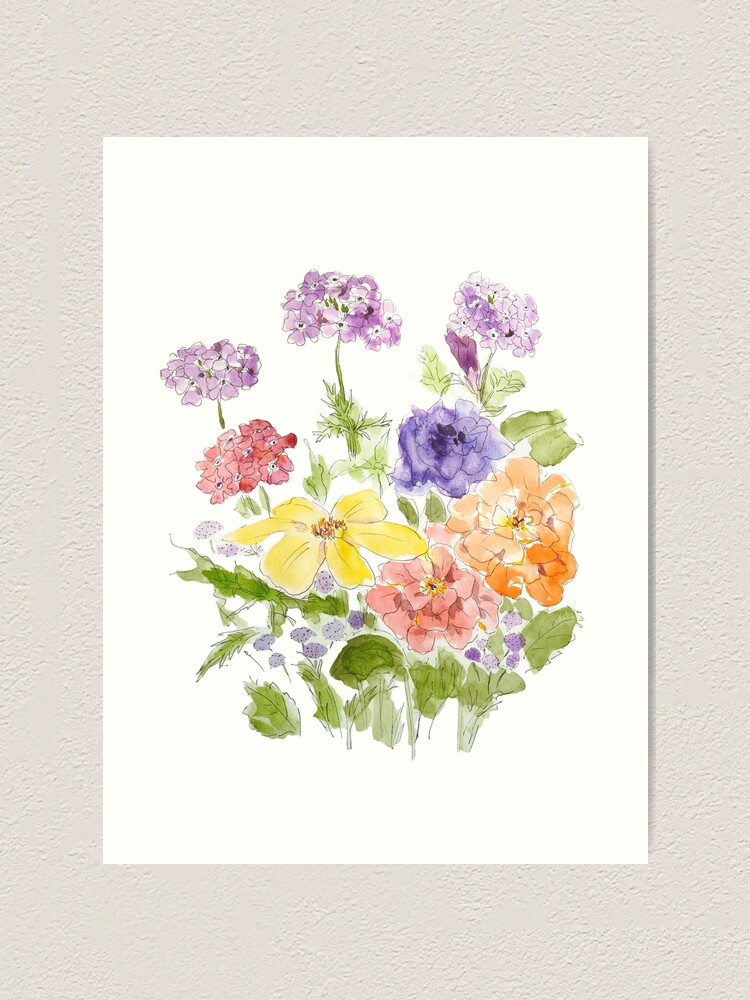The image is a detailed watercolor illustration of a diverse array of wildflowers, depicted on bright white paper. The scene likely represents an outdoor garden or field, though there's no ground depicted—just a white background. The illustration features a rich assortment of flowers in various vibrant colors, including yellow, purple, lilac, red, orange, bluish-purple, and pink, accompanied by green foliage. The composition includes a variety of flower types such as a six-petaled yellow flower, candy tuft-like purples, violet-like blooms, clusters that look like hydrangea blossoms, and possibly lantana. The foliage is equally diverse, featuring broad leaves, serrated leaves, delicate fronds reminiscent of dill, and some unopened flower buds. The illustration itself appears to be photographed against a textured, whitewashed wall. It is unframed, unmatted, and unsigned, giving it an unfinished and personal artistic touch, much like something one might find on a beautifully crafted greeting card.